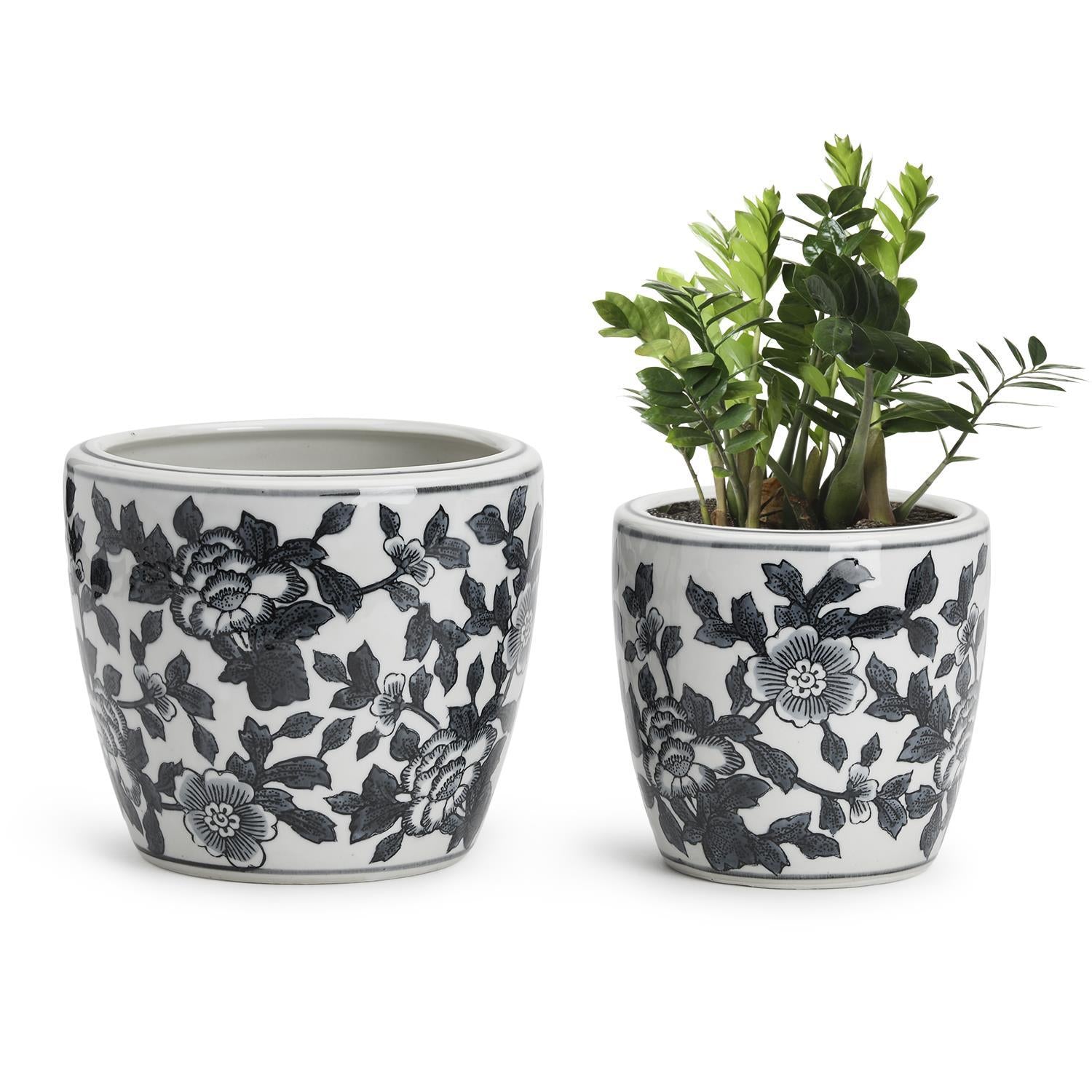In the image, two ceramic flowerpots are displayed against a plain white background with slight shading indicating the light source is from the right. Both pots are medium-sized and feature a black and white floral and leaf design that wraps around their surfaces. The pot on the left is slightly larger, with a base roughly one inch in diameter, widening to about one and a half to two inches at the top, and is empty. The pot on the right is smaller, with similar dimensions and the same detailed pattern, but contains a healthy green plant with thick stalks and long elliptical leaves, possibly a type of fern.